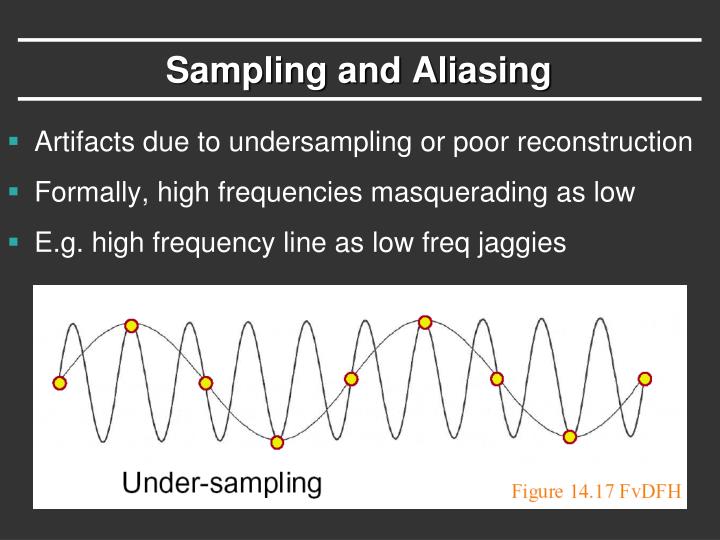The image depicts a page titled "Sampling and Aliasing" against a solid dark gray background, almost like charcoal. White horizontal lines frame the title at the top of the page. Below the title, there are three blue bullet points, left-aligned in white text, that read: "Artifacts Due to Undersampling or Poor Reconstruction," "Formally High Frequencies Masquerading as Low," and "e.g., High Frequency Line as Low Freak Jaggies." 

Occupying the bottom half of the image is a rectangular graph featuring jagged and curvy black lines resembling a sine wave, with scattered yellow dots throughout the graph. A caption below the graph states "Under-Sampling," and a red label in the lower right-hand corner reads "Figure 14.17 FVDFH."